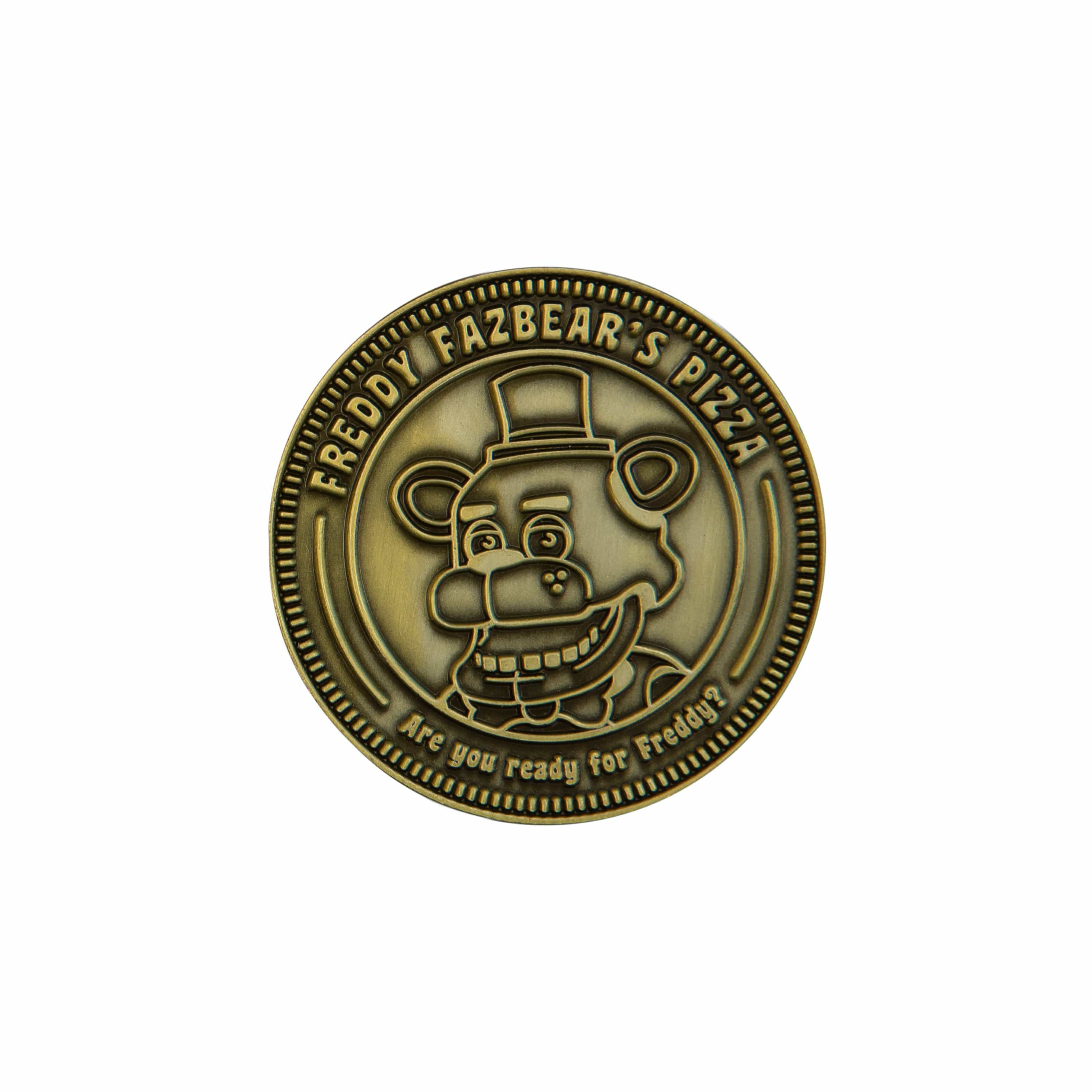This is an up-close photograph of a bronze-colored token designed for Freddy Fazbear's Pizza, reminiscent of arcade tokens used at places like Chuck E. Cheese's. The token stands out against a white background, highlighting its circular form. Along the top edge, in text shadowed with black for clarity, it reads, "Freddy Fazbear's Pizza," and along the bottom, it states, "Are you ready for Freddy?" In the center, there's an engraved image of Freddy Fazbear—a bear with a somewhat eerie appearance. Freddy sports a bowtie and a small top hat, with prominent features like round eyes, thick eyebrows, a large nose, human-like teeth, and ears sticking out. The edge of the token is adorned with small tactile lines, adding to its realistic coin-like texture. This detailed representation draws inspiration from the horror video game series *Five Nights at Freddy's*, evoking a sense of nostalgic yet creepy amusement akin to childhood arcade experiences.